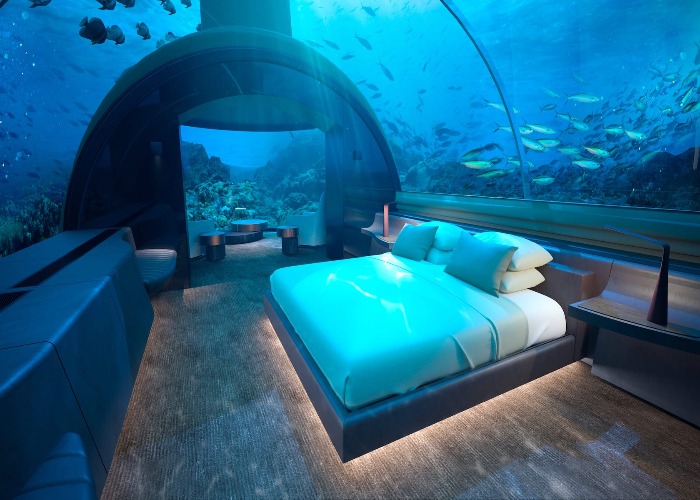This image showcases a breathtaking underwater hotel room, presumed to be an exclusive and possibly expensive destination. The room is encased in a glass enclosure, providing a panoramic view of the ocean teeming with various fish and marine life. The bed, positioned on a gray or black platform, is adorned with teal and white linens, blending harmoniously with the aquatic surroundings. To the side of the bed is a brown table with an interesting sculpture. The floor beneath is a mix of brown and white, illuminated by subtle lighting. The room features a large glass opening that offers a continuous view of the vibrant underwater world. There's a distinctive rounded metal structure around the room, possibly related to the oxygen supply, and a tower-like extension that hints at additional functional components of this unique setup. Adjacent to this room, another space with tables and seating can be seen. Above, natural sunlight filters through the water, casting an ethereal glow into the room, further enhancing the serene and immersive underwater experience.